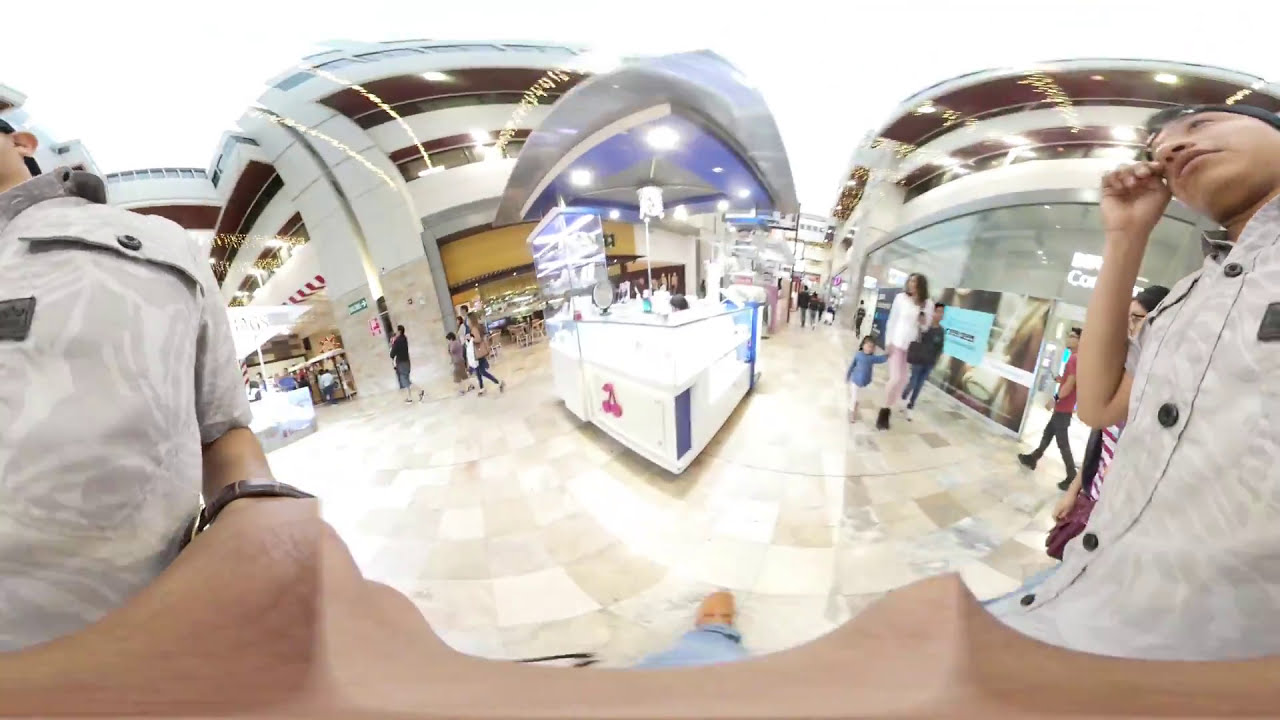The image presents a 360-degree panoramic view of a large, multi-story indoor shopping mall adorned with bold, beautiful lighting, possibly indicative of the holiday season, as Christmas lights are visible reflecting in the windows. Central to the scene is a busy kiosk, likely a jewelry or phone accessory stand with a glass display case, manned by a well-dressed individual in a beige-gray dress shirt with black buttons who is captured holding a fishbowl camera. This man appears twice due to the lens's unusual capture angles and is seen scratching his eye. Around the kiosk, a diverse crowd of shoppers, including a mother holding her daughter's hand, navigate the bustling corridors lined with stores on both sides featuring glass facades. Adjacent to the main kiosk is a small food stand, along with a small restaurant nearby with empty chairs. The overall scene is dynamic, with multiple levels of stores extending into the distance, embodying the vibrant atmosphere of this spacious, possibly Asian, shopping center.